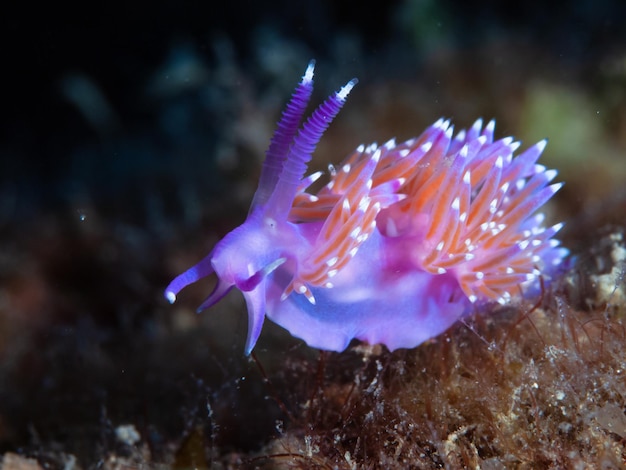The photograph showcases a striking underwater scene featuring a vibrant, slightly translucent sea slug with a captivating mix of colors. Primarily purple, the creature is adorned with spiky protrusions that exhibit a gradient from orange to purple, ending in distinctive white tips. Its tiny black eyes peer forward, and it boasts two horn-like, textured antennas that culminate in small, white, light-like tips. Around its body, anemone-like appendages add to its intriguing appearance. The entire form of the sea slug appears perched on a dark, bristled, sponge-like substance, surrounded by blurry yet similarly textured underwater elements. Red seaweed can also be seen at the bottom of the image, adding to the rich, vibrant palette of this professionally captured scene.